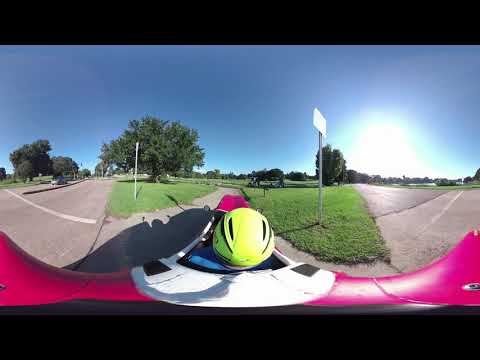This detailed photograph captures a motorist in a hot pink and white racing vehicle. The driver is positioned in the white cockpit area of the small, sit-in, motorized vehicle, reminiscent of a pedal car or go-kart, sporting a bright neon yellow helmet with black stripes and a blue shirt. The camera angle, likely from a GoPro mounted behind the driver, offers a rear view of the vehicle as it navigates the center of three parallel streets, bordered by grassy patches that separate the lanes. The sun, appearing to be just rising, illuminates the scene under a clear, deep blue sky with no clouds. Two circular mirrors are visible in front of the driver, and small street signs are situated within the grassy dividers. The backdrop suggests a rural or park-like environment, with shrubbery, grass, and a distant horizon marked by trees and an elevated, angled sign on a pole. The road appears to slightly curve to the left and right, reinforcing the impression of a raceway setting.